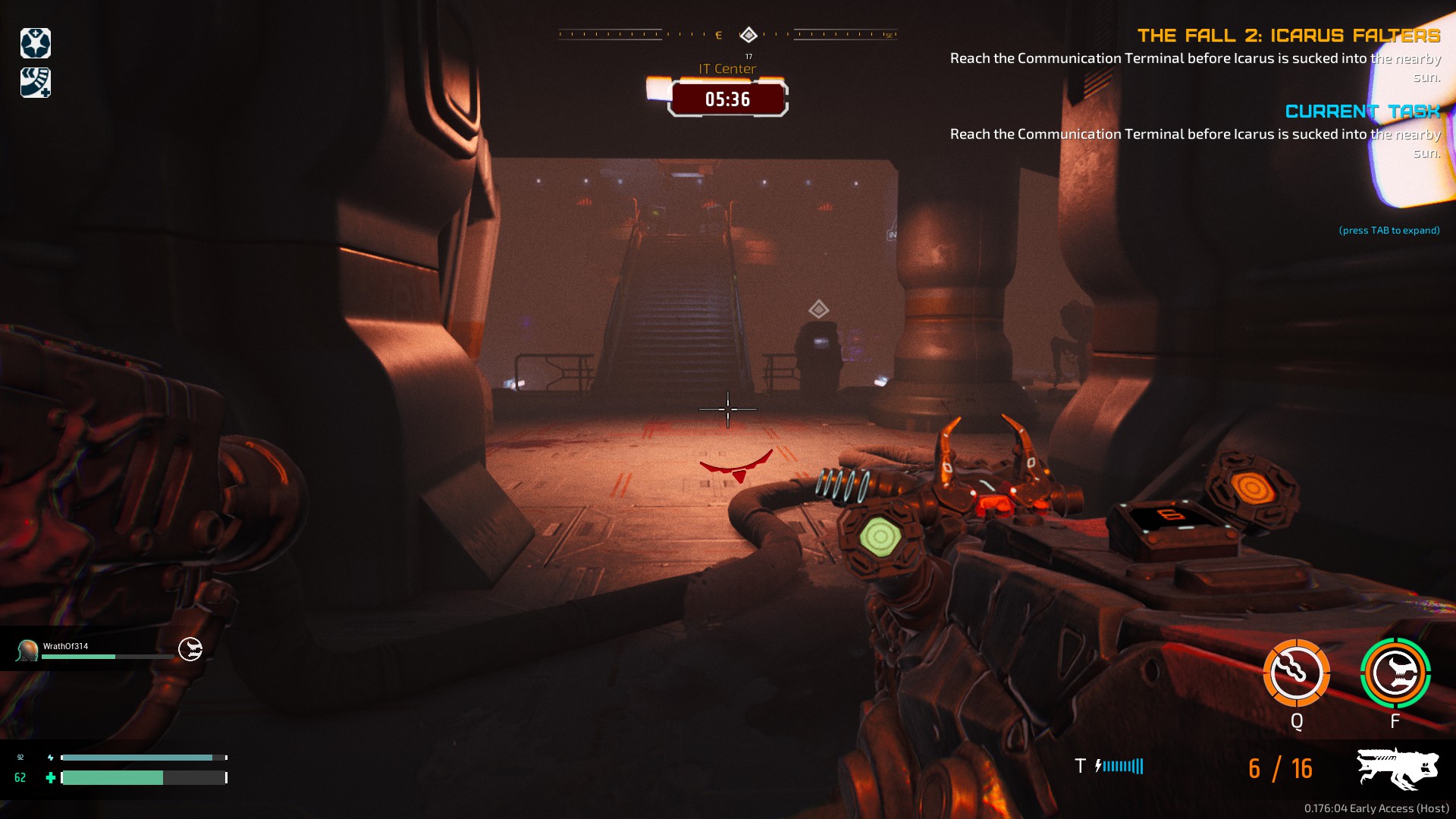In this detailed screenshot from the video game "The Fall 2: Icarus Falters," the player is immersed in a dark and ominous basement-like setting, viewed from a first-person shooter perspective. The screen depicts the player's futuristic gun, adorned with strange lighting and complex geometry, prominently in the lower right. Beside it is a HUD showing pertinent gameplay information such as health, ammo, and directional indicators, with the ammo or energy count displayed as "6 out of 16." Surrounding the player is a sci-fi corridor, complete with dim, warm orangish lighting that punctuates the otherwise gray and black tones. To the left of the scene lies another weapon, while distant stairs and floor-bound pipes contribute to the eerie atmosphere. Above the gameplay area, mission-critical text— "Reach the communication terminal before Icarus is sucked into the nearby sun"—is reiterated, underscoring the urgency of the player's task.